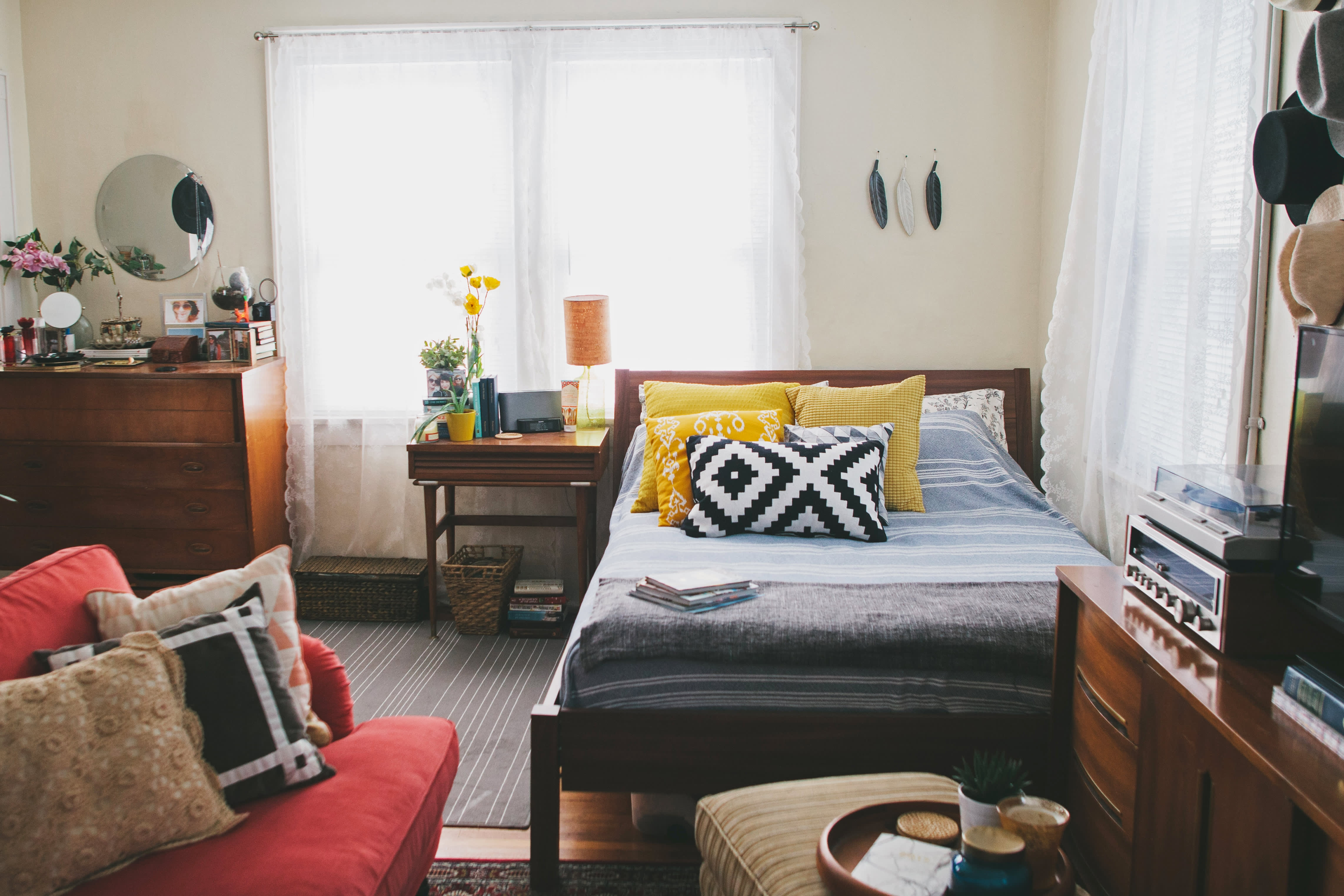The image depicts a cozy, small bedroom with white walls. The focal point is a full-size wooden sleigh bed, positioned against the right wall, adorned with a gray woolen comforter. Five decorative throw pillows embellish the bed: three yellow ones at the back and two white ones with black or brown square and triangular patterns at the front, exuding a southwestern flair. Adjacent to the bed on the left sits a wooden nightstand with a wicker waste basket underneath. This nightstand holds a pot of vibrant yellow flowers and another pot housing an aloe vera plant in a yellow pot. 

In front of a window with white curtains, which perfectly blend with the walls, is a simple brown side table. To the left of the table, positioned near the bottom left of the image, is a red suede love seat. This seat is partially visible, showing enough space for one person, and is decorated with three throw pillows: one brown, one black and white with a square pattern, and one white.

On the far left, a wooden dresser topped with a pink flower in a pot sits under a round mirror mounted on the wall. Above a small TV to the right, three hats hang—one tan, one black, and one gray, adding a touch of personality to the room. This intimate setting suggests it could be part of a studio apartment, welcoming with its warm and vibrant decor.